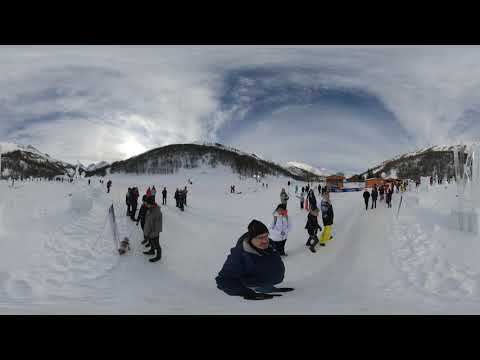In the image, a distorted fisheye lens effect captures a crowded snowy landscape, lending a rounded curvature to the scene. Directly in the foreground sits a man, a Caucasian male, donning a black hat and a navy blue winter jacket, appearing legless due to the distortion. The ground is blanketed in snow, stretching as far as the eye can see. Multiple people are scattered across the snow-laden terrain, dressed in full winter gear, and potentially preparing for sledding or skiing. Among them, a woman in a white jacket stands out, as well as a group with a dog on a leash to the left, although their details are blurred and indistinguishable.

In the distance, gently rolling hills dotted with green pine trees rise, partially covered in snow. The sky above transitions from a clear blue on the right to thick cloud cover at the top and center, creating a duality of bright sky and overcast ambiance. A particularly bright spot near the left of the hills suggests the sun peeking out from behind the clouds, contributing to the surreal, curved arcs of the sky caused by the lens distortion.

The scene's comprehensive view, possibly from a 360-degree image stitched into a flat frame, encapsulates people congregating around what appears to be a ski slope or winter recreational area, with signs and pathways visible amidst the snow. The combination of elements—clear skies, cloud cover, vivid winter attire, and a snowy, scenic backdrop—paints a vivid picture of an outdoor winter wonderland, bustling with activity.